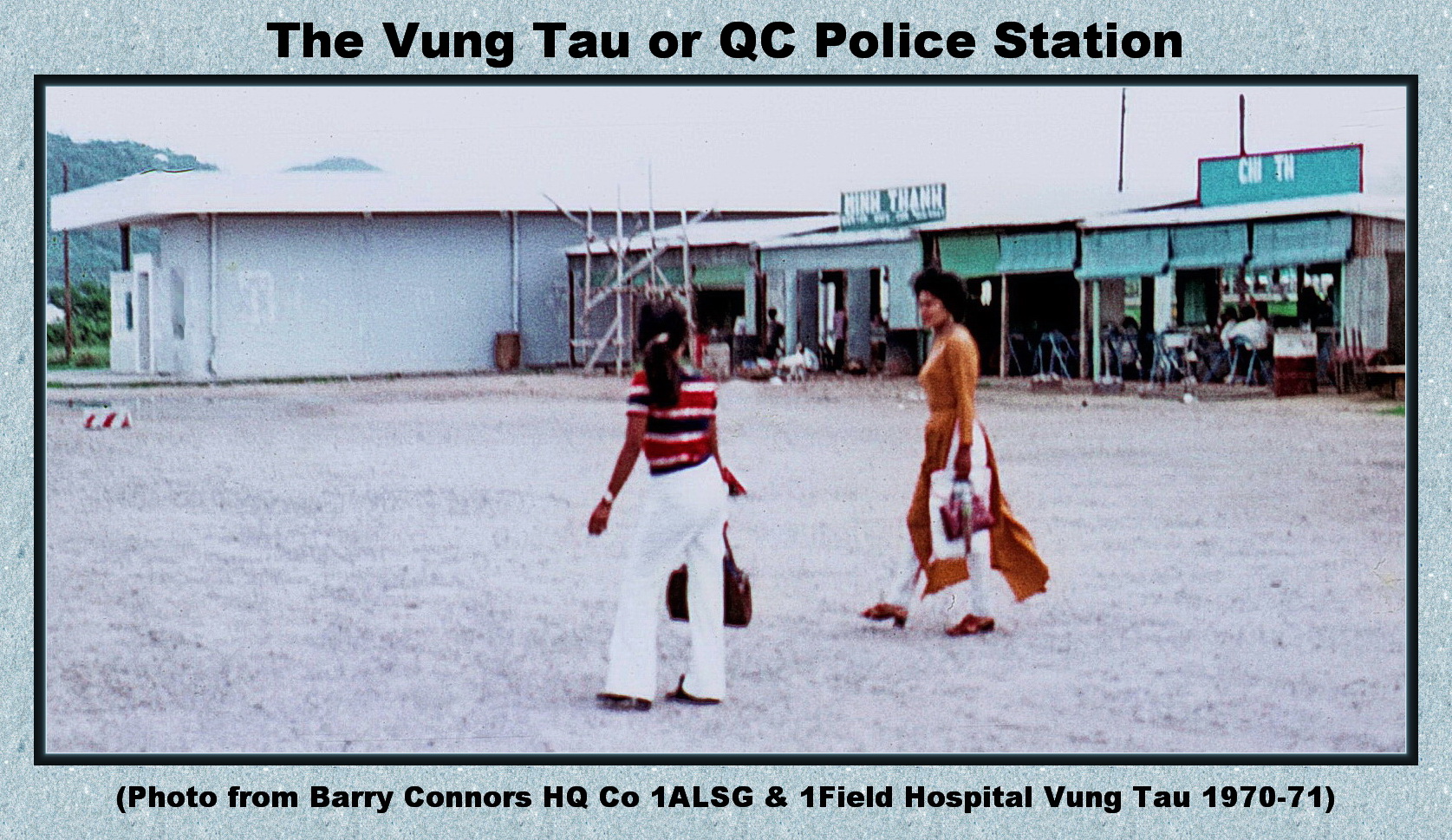The image is framed by two distinct borders, providing a structured and eye-catching presentation. The outer border is a light blue color, while a darker blue inner border adds depth and emphasis to the central photograph. At the very top of the light blue border, black text reads "Vung Tau QC Police Station." At the very bottom, black text in parentheses states, "Photo from Barry Connors, HQ, CO 1ALSG and One Field Hospital, Vung Tau, 1970-71."

The central photograph captures a moment in a gravel parking lot where two women are walking. The background features two metal sheet buildings: a green building with roll-up curtains that are currently raised, and a white rectangular building. The green building's open curtains suggest activity, while the white building stands alongside in a more understated presence. This photograph provides a glimpse into the scene at the Vung Tau QC Police Station during the specified period.